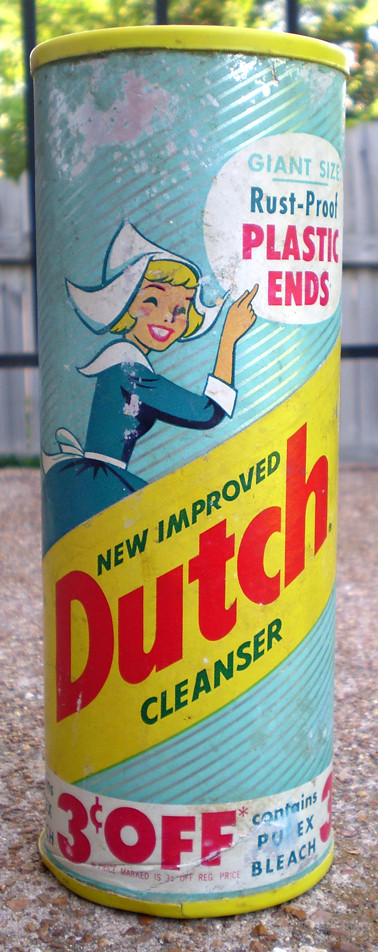This color photograph, taken outdoors during the day, showcases an old, vintage canister of Dutch Cleanser placed on what seems to be a gravel road with a distinct reddish hue. The canister, reminiscent of a Comet cleanser container, is predominantly light blue with diagonal silver stripes running from top to bottom. Prominently featured on its front is an image of a Dutch woman dressed in blue and white attire, with blonde hair, pointing towards a white sign. The sign reads, "Giant Giant Size Rust-Proof Plastic Ends.” Just below this, a yellow banner with the text "New and Improved Dutch Cleanser" is displayed. Near the bottom, a label indicates “Three Cents Off” and mentions that the product “Contains Purex Bleach.”